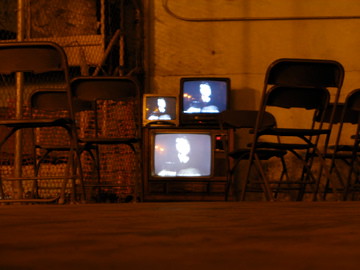This photograph captures a dimly lit, possibly nighttime, outdoor scene featuring an impromptu viewing area set against a stone wall and floor, bathed in an orange light. At the center are three television sets: an old, vintage console TV at the bottom with a prominent front display, and two smaller TVs stacked on top of it. The left TV is small and silver-colored, while the right one is slightly larger and black. All three TVs display the same indistinct, blurry image of a face against a dark backdrop. Surrounding the televisions are metal folding chairs, suggesting a makeshift arrangement, possibly indicative of a basement-like environment, complete with a presumed basement window in the upper left corner. The area is bordered by a metal fence to the left. The overall color palette transitions from yellowish-brown in the foreground to a light butterscotch shade in the background.